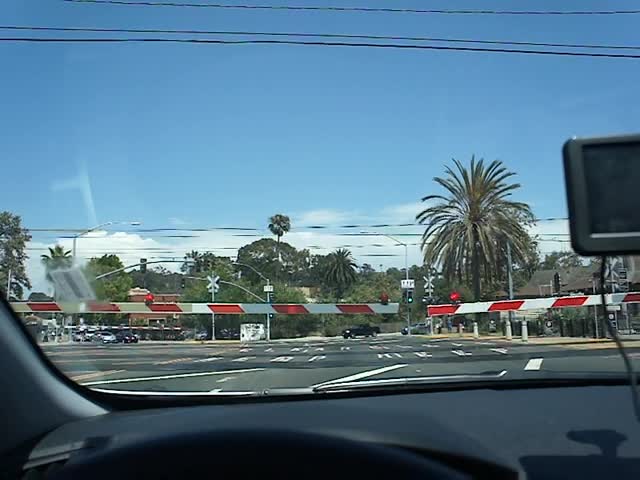The photograph captures a vivid scene from the driver's seat of a car. The black dashboard spans the bottom of the image, though the steering wheel is not visible. Gazing through the vehicle's windshield, a picturesque blue sky adorned with wisps of clouds stretches across the horizon. Dominating the center of the image, a red and white railroad crossing stands tall, indicating the proximity of a railway track. To the top right, a black square device, possibly a GPS unit, is mounted discreetly. In the midst of this urban setting, a cluster of palm trees rises, flanked by lush green foliage. Overhead, black telephone wires crisscross the sky. The road ahead is clearly marked with white pavement lines, leading up to an intersection on the left where traffic lights and indistinct brick buildings are faintly visible in the distance. The scene is a detailed snapshot of a tranquil moment paused at a railroad crossing, with layers of both natural and urban elements blending seamlessly.